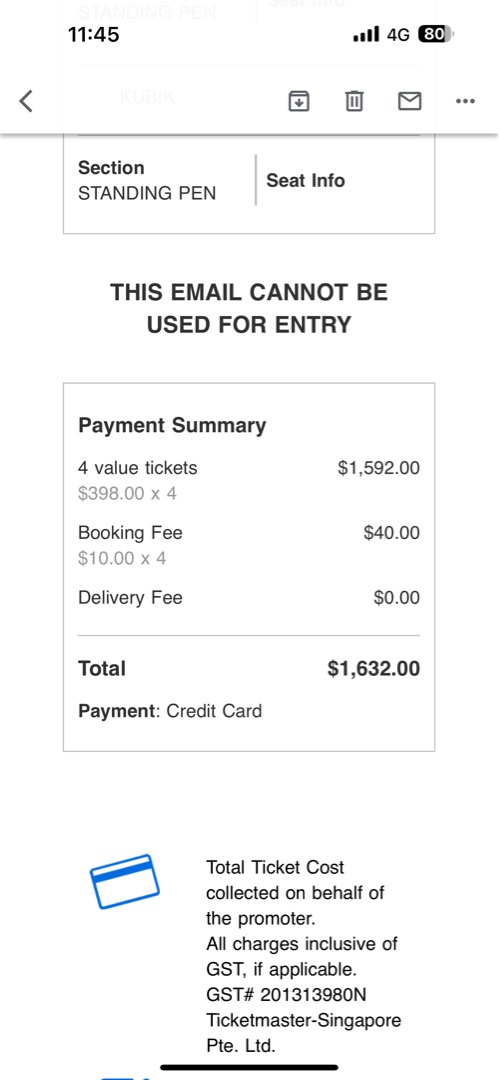**Detailed Caption:**

A cell phone screenshot with a predominantly white background. At the top left, the time reads "11:45" in black text. On the top right, icons indicate cell phone signal coverage, 4G connectivity, and a mostly full battery displayed in black with an "80" in white text, indicating 80% battery life. 

The next line features a back arrow pointing left, and on the right side, there are icons for download, trash, envelope, and three vertical dots. Below this is a gray dividing line, after which the white background continues.

Within a gray box on the left side, "Section Standing Pen" is written in black text. Underneath is a small horizontal black bar followed by the text "See Info" also in black. Below that, in bold white text, it states "This email cannot be used for entry." 

Following this, in a square gray area, "Payment Summary" is written in black text. Detailed ticket information follows:
- "Four tickets" on the left, with "1,592" on the right.
- Below, in gray text, "398x4" indicates the unit price of the tickets.
- Next, "Booking Fee" is listed in black, amounting to "$40" with "10x4" shown in gray beneath it.
- "Delivery Fees" are marked as "$0."

The total cost is calculated at "$1,632," with the payment method specified as "Credit Card." 

A small white space separates this section from a blue credit card icon, which indicates that the total ticket cost includes all charges and GST. 

At the bottom, there’s a note in black text mentioning "Ticketmaster Singapore PTE. LTD," providing some context about the booking and a subtle commentary that even Singapore deals with Ticketmaster's service.